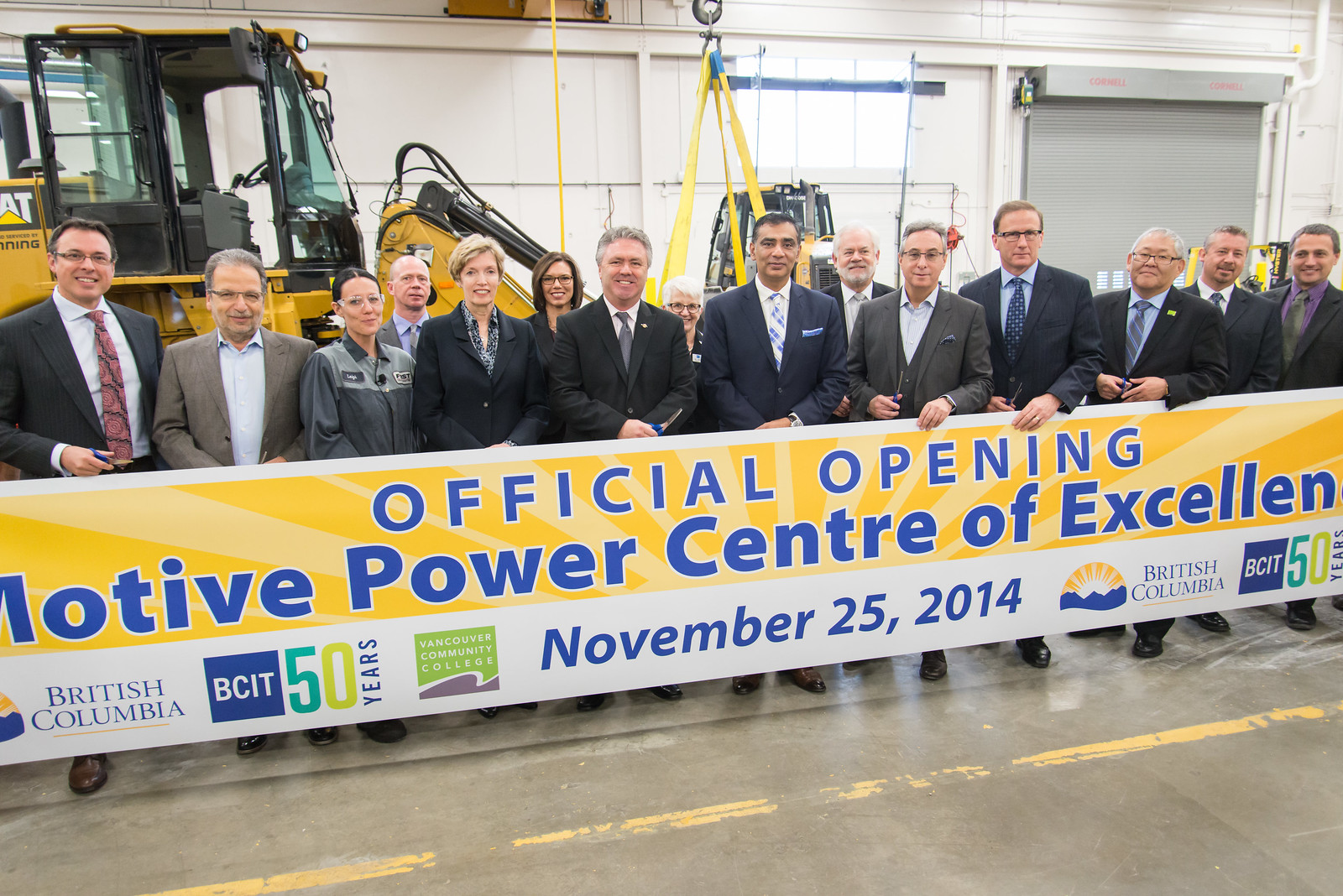A group of official-looking individuals, dressed primarily in suits, stands together in an industrial facility for a photograph. They are positioned behind a large banner that reads, "Official Opening Motive Power Center of Excellence," with additional text indicating "British Columbia, BCIT, 50 years, Vancouver Community College, November 25, 2014." Behind the group, various industrial equipment, including a forklift and a large Caterpillar backhoe, are visible, reinforcing the setting as a warehouse or factory. The backdrop includes gray concrete flooring with a worn yellow line and various shades of yellow, blue, green, black, gray, white, and red adding visual interest to the scene. The image captures a momentous occasion, likely taking place indoors in the middle of the day, characterized by the official attire of the attendees and the formal tone of the event.